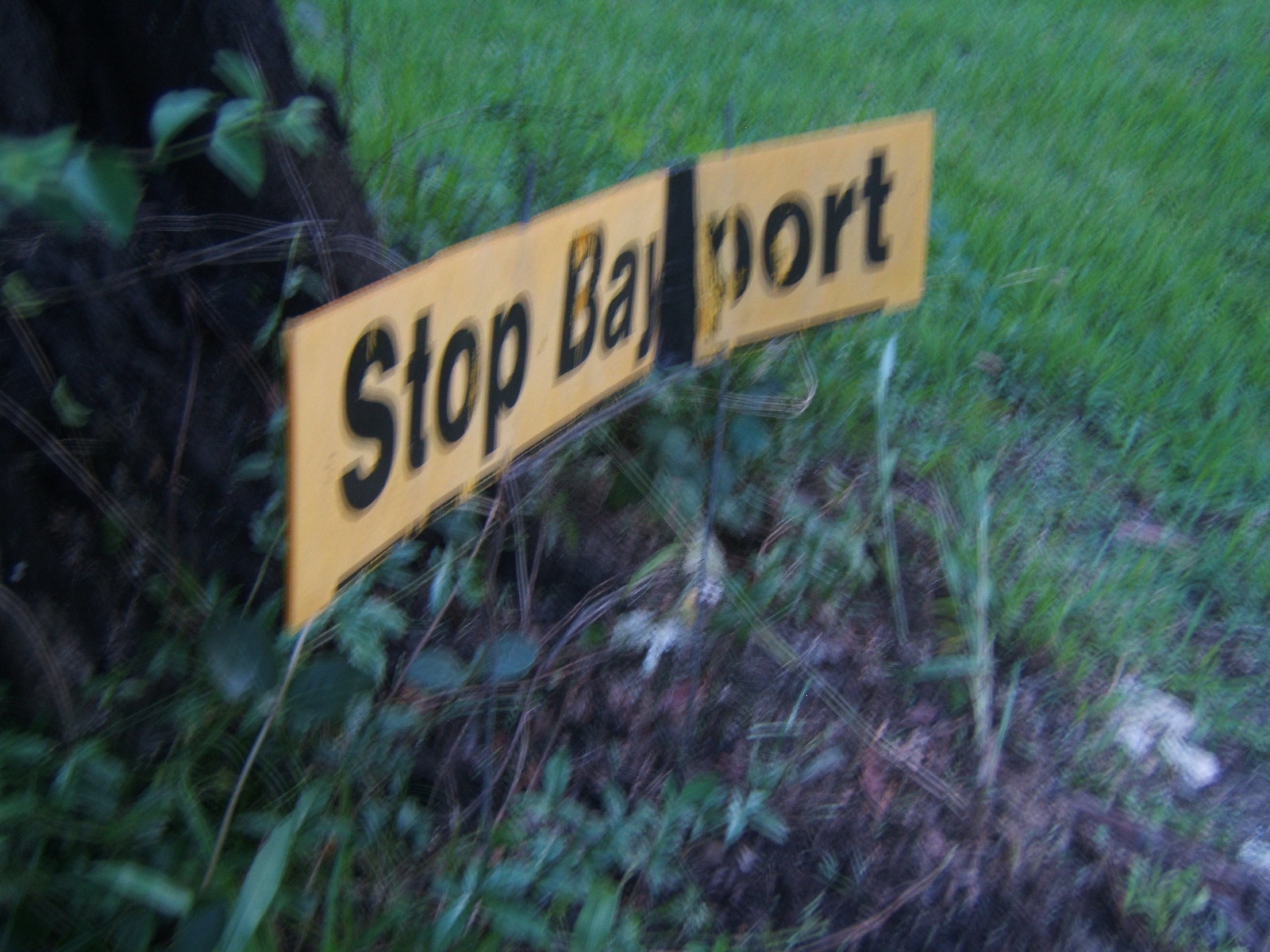In this close-up image, a small, rectangular yellow sign is prominently featured. The sign, mounted on metal stakes that are driven into the ground, bears the text "STOP BAYPORT" in bold black letters. Notably, the sign is broken between the letters "Y" and "P" in "Bayport," creating a noticeable gap. The background in the top right corner of the photo showcases a lush expanse of grass, while the bottom left corner includes the base of a tree with visible roots and surrounding weeds. The sign is positioned directly at the base of the tree, blending into the natural elements of its surroundings.